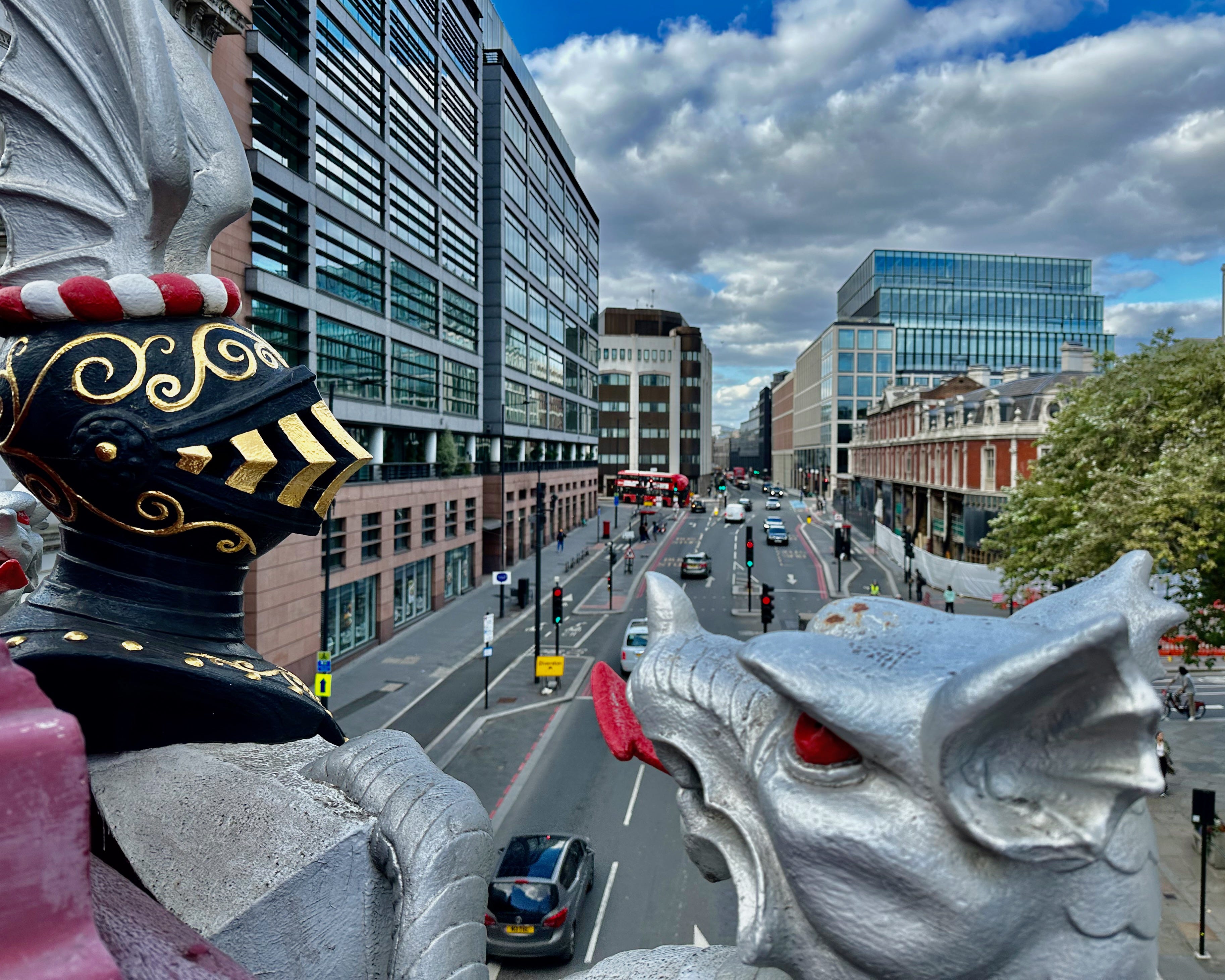In the foreground of this vibrant city street scene, a striking statue captures immediate attention, featuring a knight clad in shiny silver armor with a black and gold helmet alongside a silver dragon with vivid red eyes, a protruding red tongue, and intricate features reminiscent of a mythical creature. The photo, taken during the day under a clear blue sky dotted with white, puffy clouds, showcases a multi-lane road flanked by tall, modern buildings predominantly constructed with large glass windows, interspersed with some light brick buildings. Cars travel in opposite directions on either side of the road, hinting at a non-U.S. location, and a red double-decker bus is discernible in the far left background. Numerous pedestrians can be seen walking along the pavements, adding to the bustling atmosphere. Slim black poles holding streetlights and electric signs punctuate the streetscape, while occasional trees add a touch of greenery to the urban environment.